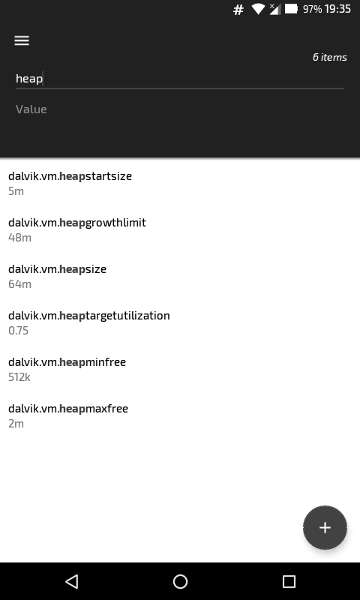The image captures a screenshot taken on an Android phone, evident from the portrait orientation and distinct UI elements like the Wi-Fi, data, battery icons, and the time displayed on the top right. The navigation bar displays familiar Android symbols: a back arrow on the left, a circle in the center, and a square on the right. The app interface shown has a hamburger menu in the top left and a search bar at the top with the query "heap" entered. Below the search bar, the screen is divided into six items labeled with terms such as "dalvik.vm.heapstartsize," indicating specific Android configuration values. Each item is accompanied by varying numerical values (e.g., 5m, 40m, 0.75, 512k), possibly representing memory sizes or heap specifications. The detailed components suggest that the user is navigating through technical settings or developing an application, particularly focusing on Dalvik VM configurations rather than engaging in regular user activities.